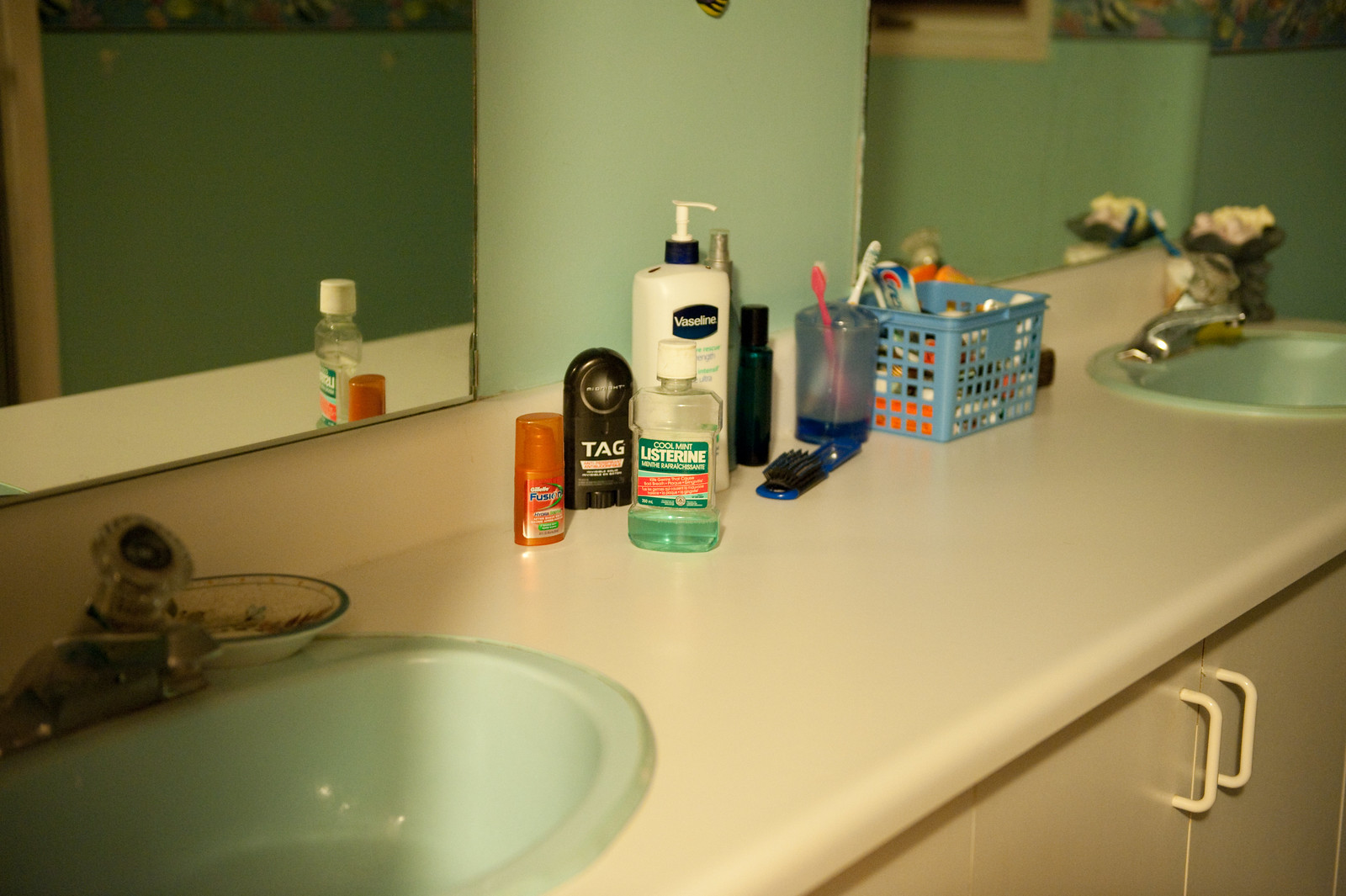The image depicts an older-style bathroom featuring two greenish sinks set against similarly colored walls. These dual sinks, reminiscent of a his and hers setup, are integrated into an off-white countertop that matches the off-white cabinets below. Above each sink is a dedicated mirror, with a common space situated in between. On the countertop, various toiletries are visible, including deodorant, Crest toothpaste, Listerine mouthwash, and hand lotion. To the right, there seems to be a decorative item that possibly serves as a soap holder, while another soap dish with a small piece of soap is positioned to the left. The bathroom features older fixtures and approximately a foot or two above the sinks, a green wallpaper with a floral border further emphasizes the vintage aesthetic.